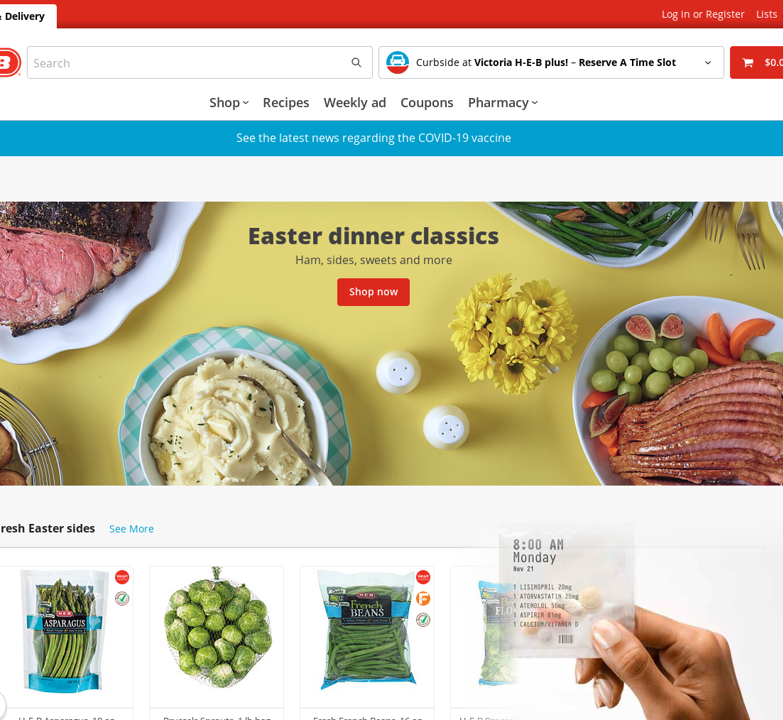The screenshot displays the H-E-B Grocery Store's online shopping website, specifically the curbside service page for the Victoria H-E-B Plus location. At the very top of the page, there's an option to reserve a time slot for curbside pickup. To the upper left, a partially visible tab for delivery services is cut off. On the upper right, there's a "Log In or Register" button, visible but positioned above an obscured logo. Below this, an empty shopping cart icon is displayed, showing a total of $0.00.

Centrally featured on the page is a promotional banner that reads "Easter Dinner Classics: Ham, Sides, Sweets and More," showcasing various Easter-themed food items. Below the promotional ad, there is a partially visible section titled "Fresh Easter Sides," highlighting vegetables like asparagus, Brussels sprouts, and green beans, along with another indeterminate item.

Above this section, a stock image is shown of a woman's hand holding what appears to be prescription medications. The footer of the page and specific product details, along with brand names for the vegetables, are cut off and not visible in the screenshot.